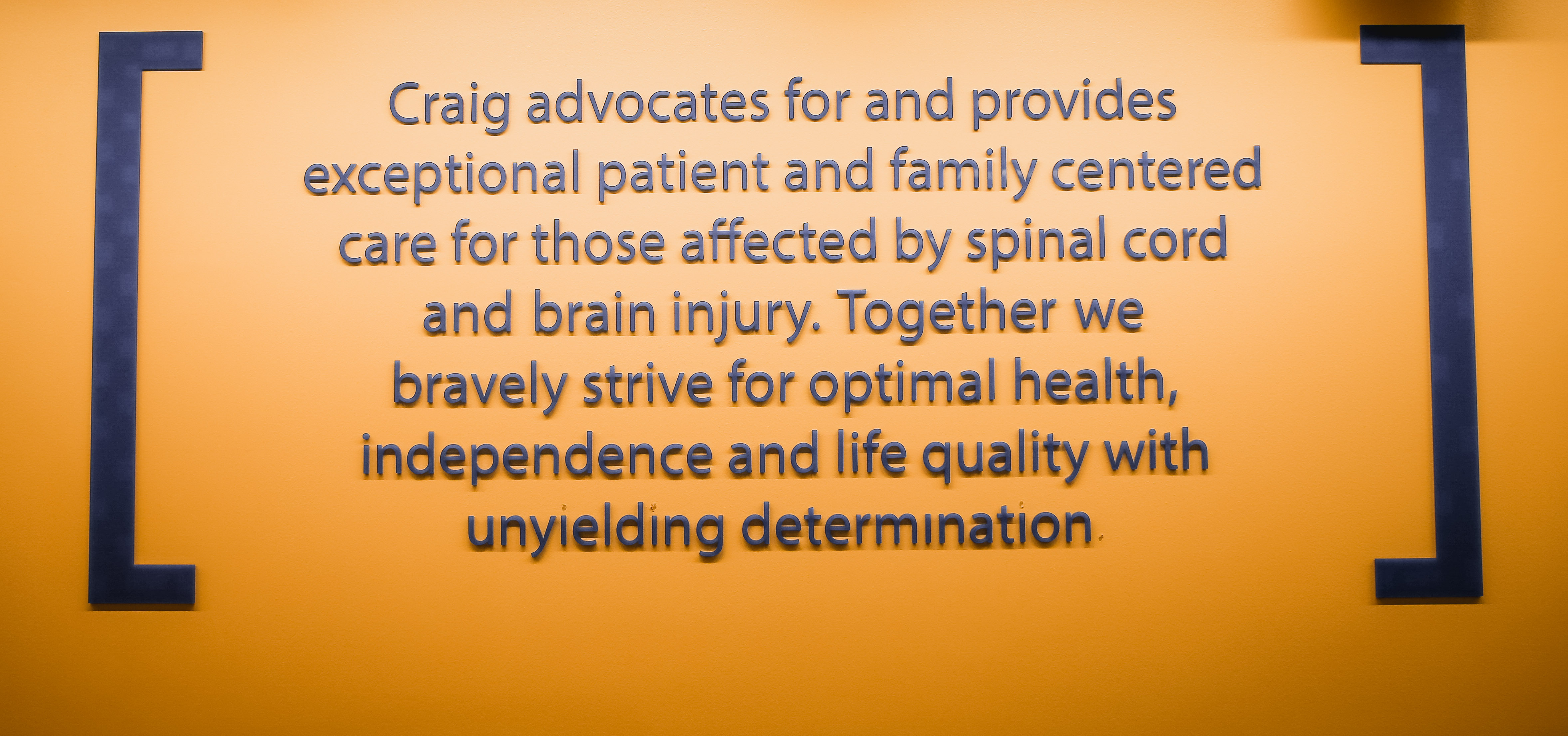The image is a horizontally aligned rectangle featuring a solid orange background that transitions into a gradient with darker edges and a lighter central area. It showcases a central block of text framed by two thick, dark blue brackets on either side. The text, written in an easy-to-read dark blue font, reads: "Craig advocates for and provides exceptional patient and family centered care for those affected by spinal cord and brain injury. Together we bravely strive for optimal health, independence, and life quality with unyielding determination." The lighting in the image enhances the central text, possibly due to camera angle and lighting conditions, making it stand out more prominently against the orange background.